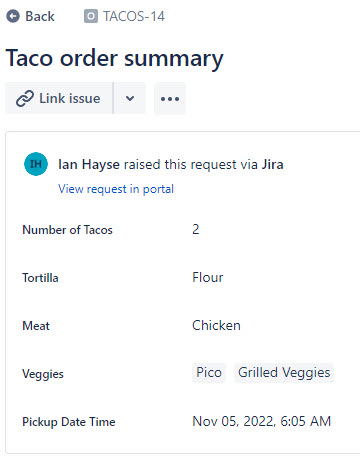Screenshot of a mobile phone screen showing a taco order summary. At the top of the screen, a charcoal-colored arrow points to a section labeled "Tacos," rendered in a matching charcoal or gray font. Next to this label, the word "tacos" appears again in a lighter gray, accompanied by the number "14," indicating that 14 tacos have been ordered. Below this section, the heading "Taco Order Summary" is displayed in bold black lettering. 

Adjacent to the order summary are the words "Link Issue" and a dropdown menu indicated by three vertical dots. Beneath these elements, a blueish-teal circle with the initials "IH" signifies that Ian Hayes requested the order via the Gyra platform. A clickable blue link that reads "View Request in Portal" is provided for additional details.

The order summary lists the specific details of the taco order:
- Quantity: 2 tacos.
- Tortilla: Flour.
- Meat: Chicken.
- Vegetables: Pico de Gallo and grilled veggies.
- Pickup Date and Time: November 5th, 2022, at 6:05 AM, indicating an early morning pickup time.